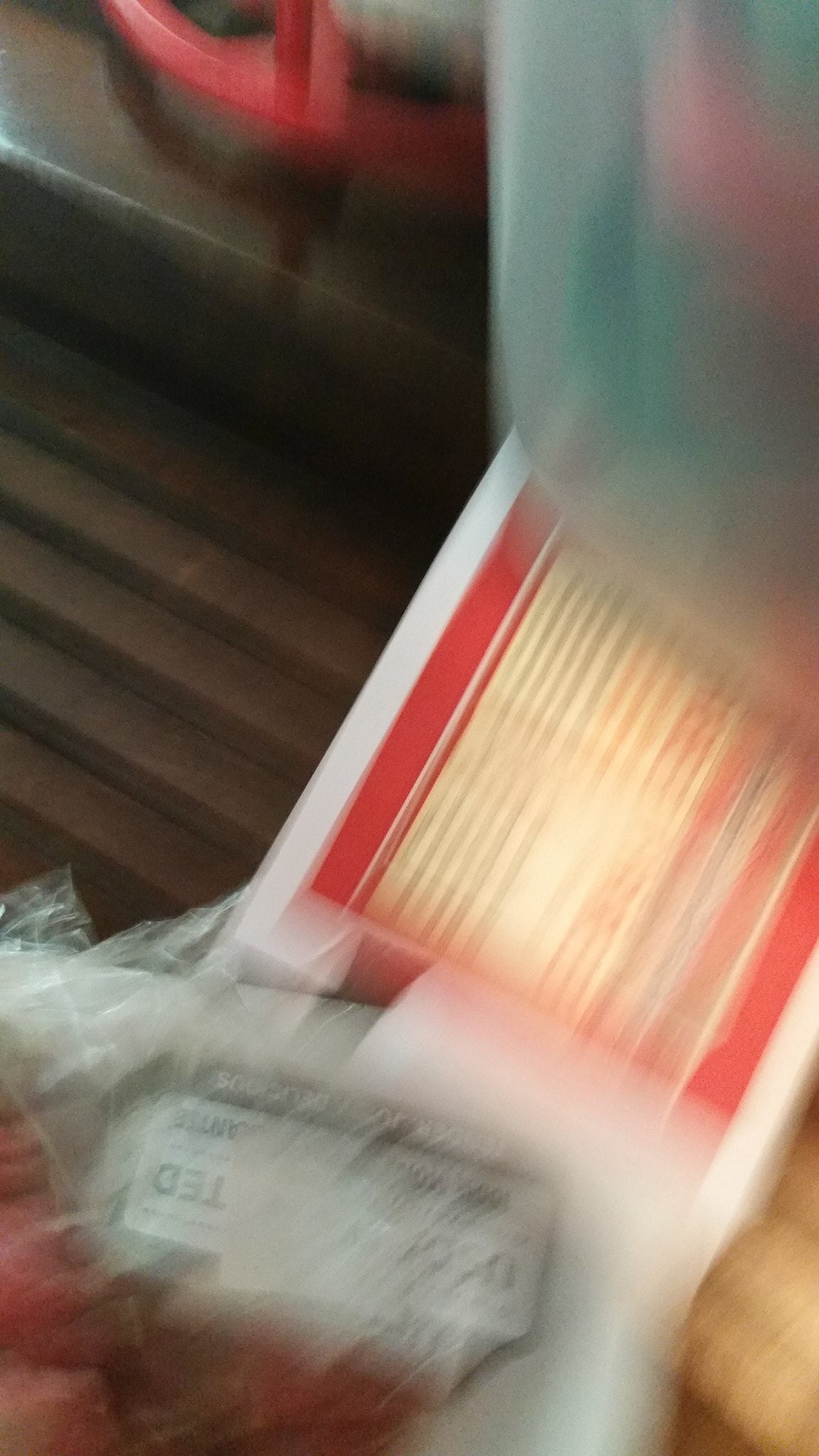In the image, an indistinct, blurry photo seems to reveal a rectangular object that might be either a menu or a paper container. Its exterior features an outline in white followed by a red border. The interior section, which presumably contains text, appears mottled with hues of yellow and blue. The object is lying on a brown surface that could either be a carpet or a floor, suggesting the setting might be indoors. All other details in the image remain unclear due to the overall blurriness.